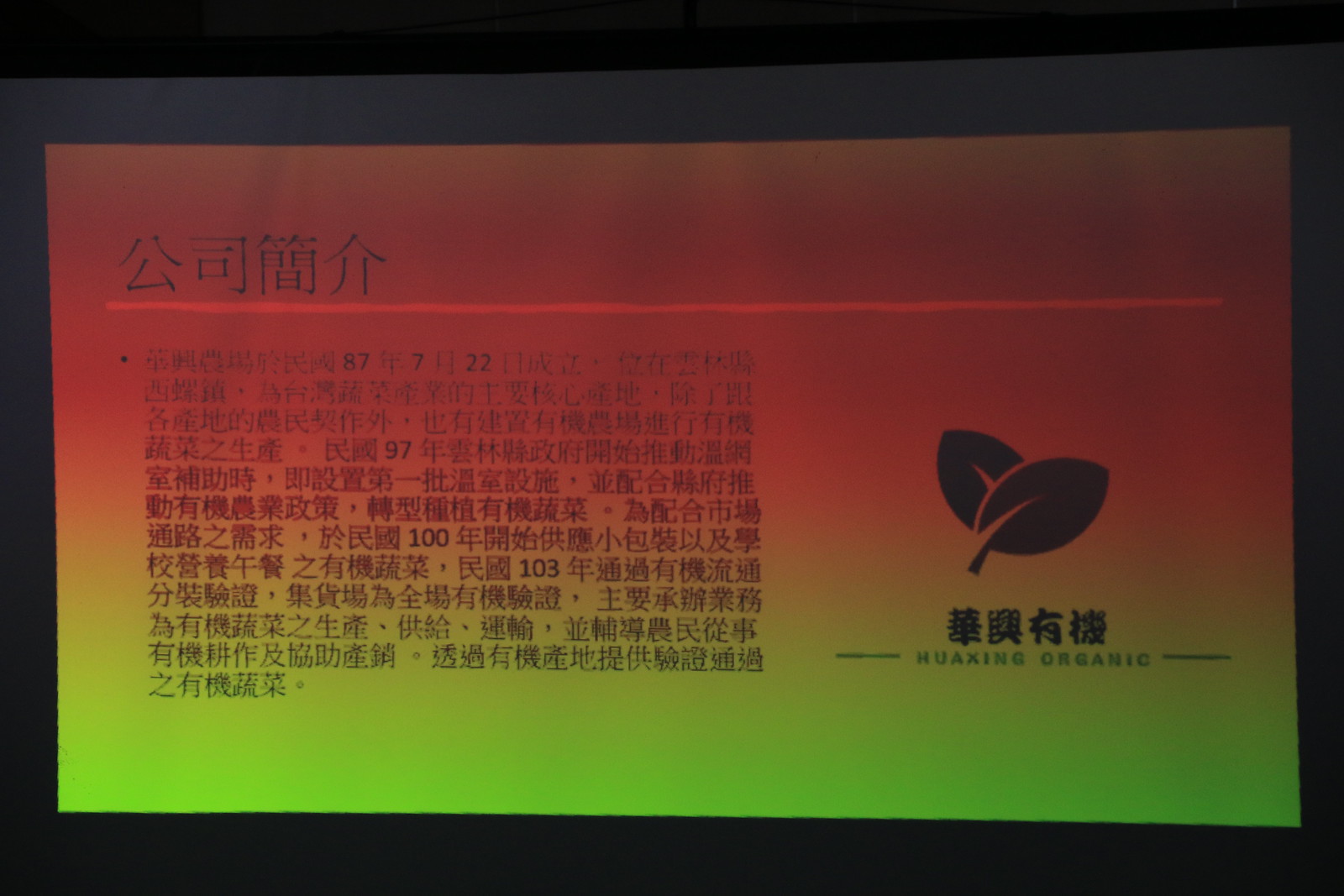The image is a PowerPoint presentation slide showcasing a Chinese company, predominantly featuring traditional Chinese characters. The slide has a vibrant gradient background transitioning from red to green hues, framed with a black border. At the top of the slide, there is prominent black text, while additional text continues along the left side towards the bottom. The slide also includes numerical details: 87-722-97100-103.

On the right side of the slide, a company logo featuring a leaf emblem is present, with the company's name, "Huaqing Organic," positioned below it in dark green text. This company, established on July 22, 1987, initially collaborated with local farmers and pioneered one of the country's first greenhouses. It specializes in organic food production, packaging, and distributing small packaged foods and school lunches. Additionally, there are pencil drawings of a tree and various house shapes adjacent to the logo.

Overall, the detailed presentation underscores Huaqing Organic's long history and commitment to organic farming and food distribution.